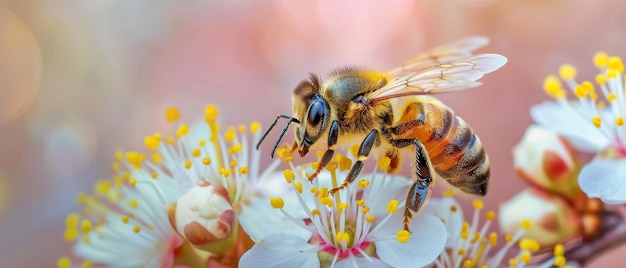The image is a detailed close-up of a bee, likely a bumblebee, engaged in pollination. The bee, characterized by its yellow body with black stripes and black legs, stands prominently in the center of the photo. It features noticeable eyes and translucent wings extended from its head. The bee is perched on a flower with white petals that have hints of pink and thin white filaments ending in tiny yellow knobs. Surrounding the focused central flower are other slightly blurry white flowers, with one bud visible to the left. The background features a mix of soft, blurry colors, including green, pink, and blue, contributing to a dreamy, almost ethereal ambiance.